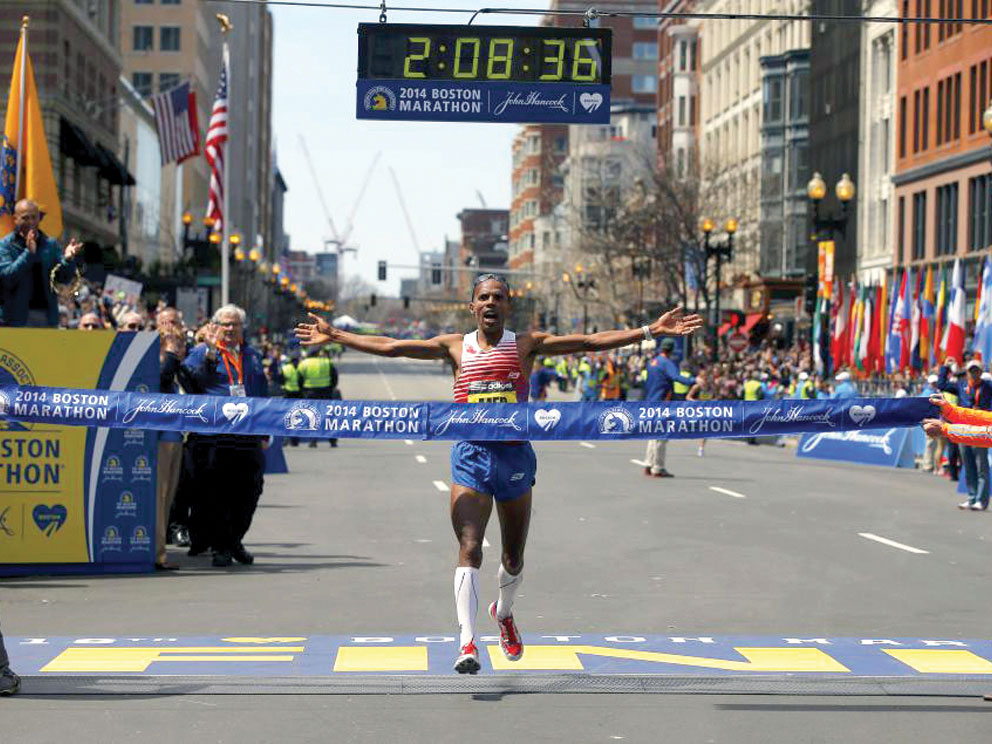In this detailed image capturing the triumphant moment of the 2014 Boston Marathon, a black man with short hair crosses the finish line triumphantly, his arms outstretched as if embracing victory. He is wearing blue shorts, white socks, and red shoes paired with a gradient white and red shirt. The blue ribbon he passes through reads "2014 Boston Marathon," and it's held on either side by people, symbolizing the finish line. Above him, suspended on a cable, is an LED timer displaying "2:08:36" in green digits, with a blue section beneath it listing "2014 Boston Marathon" and sponsor logos, including the prominent John Hancock logo. 

The bustling city street, paved with asphalt, is lined with high-rise buildings and spectators who cheer the runners on. On the right side, numerous flags from at least 30 countries intermingle with the crowd, adding a vibrant, international atmosphere to the event. Additionally, the scene includes a US flag and distinctive orange flags flanking the background, though their purpose is unclear. The atmosphere is charged with excitement and a sense of accomplishment as the runner races towards the finish line, framed by the lively street and enthusiastic onlookers.